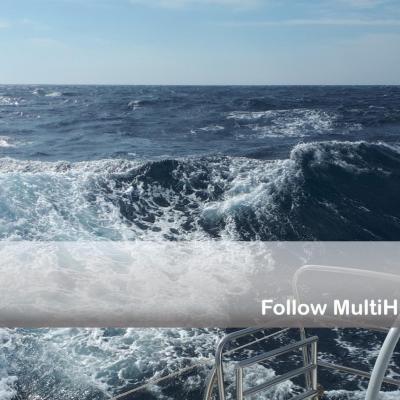The image captures a vast, deep blue ocean under a light blue sky with thin white clouds. The horizon spans the top quarter of the square frame, delineating the sky from the choppy, dark blue ocean waves that exhibit patches of white foam as they crash and merge. In the bottom right corner, metal railings indicative of a boat are visible, adding context to the perspective of the photograph. Additionally, a semi-transparent light gray banner extends across the bottom portion of the image, featuring white text that reads "FOLLOWMULTIH."